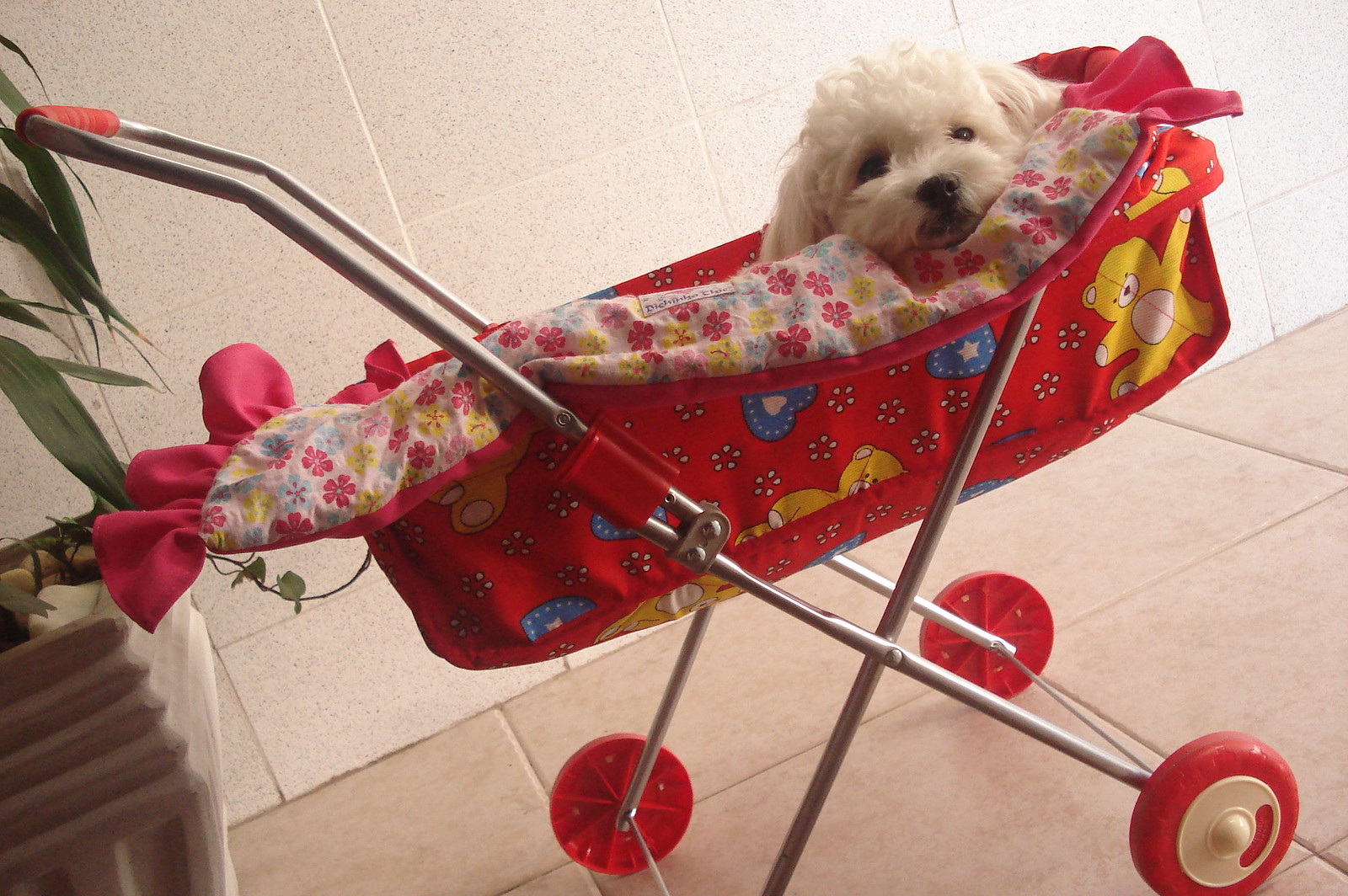The photograph captures a vibrant scene inside a well-lit building with peach-colored tiled floors and speckled peach walls with white accents. In the corner, a green potted plant rests in a brown pot. The focal point of the image is a small, fluffy white dog, possibly a poodle, comfortably nestled in a red baby stroller adorned with teddy bear illustrations and blue hearts with stars. The stroller features a shiny metal frame, red handle, and red wheels with white rims. The dog's head peeks out from the right side of the stroller, which is draped with a colorful blanket patterned with red, white, and blue flowers and fringed with red trim. The entire scene appears bright, indicating ample natural light, with no humans present in the frame.